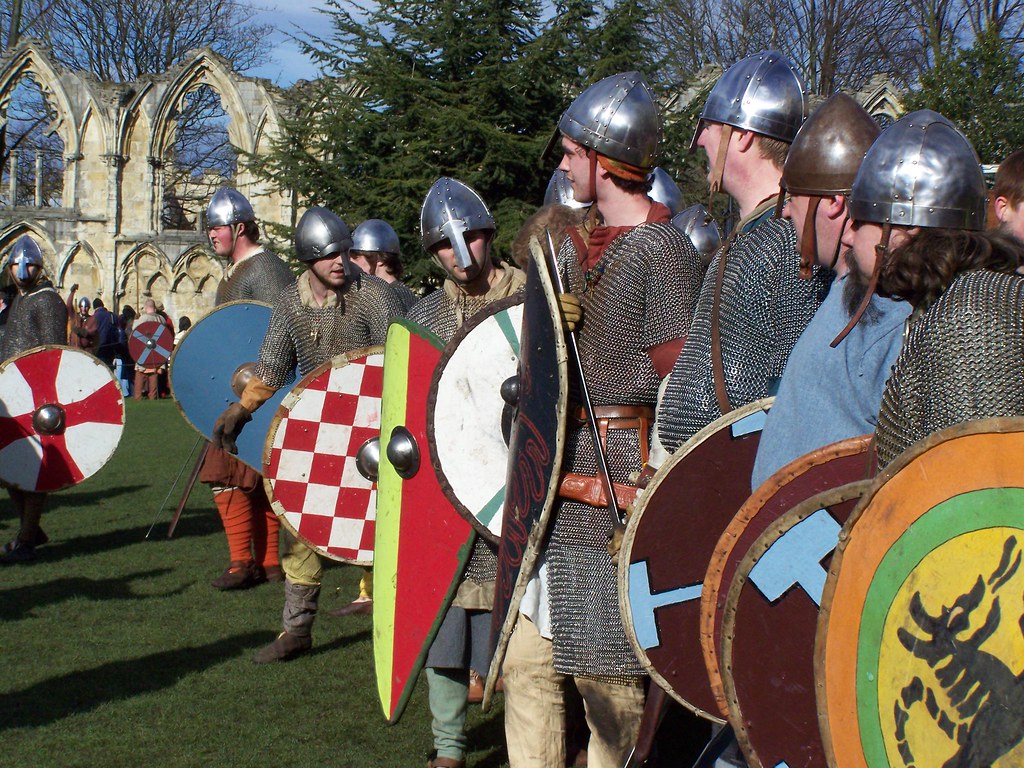On a slightly cloudy, sunny day, this outdoor scene captures a reenactment set in front of a partially dilapidated building with large arches, resembling a medieval church. The ground is covered in green grass, and the landscape includes both deciduous trees without leaves and vibrant evergreen trees. Dominating the foreground is a line of young men, possibly in their mid-20s, dressed as medieval knights. They wear elaborately detailed chain mail or old British army-like outfits, complemented by silver metal helmets with nose protectors. Each of them bears a distinct brightly colored shield, adorned with various designs such as animals and traditional red and white patterns. Their gear includes medieval shoes, gloves, and swords, contributing to the vivid historical atmosphere. In the distance, more figures in similar attire can be seen near the ancient structure, further emphasizing the immersive, period-specific setting.